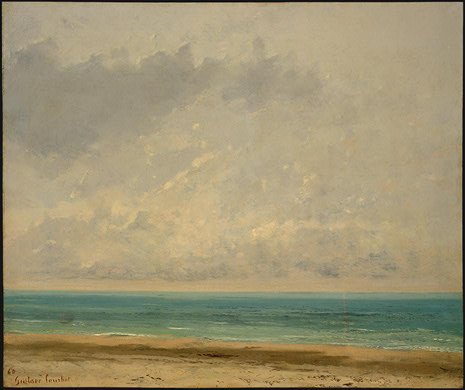This painting depicts a serene, uninhabited beach under a vast, overcast sky. The composition is set on a square parchment, emphasizing a tranquil outdoor scene devoid of any life or man-made structures. 

The beach occupies a small portion at the bottom of the image, characterized by light brown sand interspersed with darker streaks, giving a flowing, multishade texture. Approximately one-tenth to one-eighth of the painting is the sand, transitioning smoothly into the calm ocean.

The ocean itself is captured in the middle portion of the painting, roughly covering the next two-tenths to two-eighths of the canvas. It features a blend of aquamarine tones near the shore and deepening to darker blues towards the horizon. Small waves near the beach add subtle detail to the otherwise calm waters, enhancing the peaceful atmosphere.

Dominating around 70-80% of the painting is the sky, portrayed in a range of grays to off-whites with varying densities of clouds. The clouds closer to the horizon appear lighter, creating a gradual transformation to darker shades toward the top of the painting, implying a potentially overcast or post-creation scene where nature is untouched.

The artist's name is inscribed in the bottom left corner as S-U-C-K-A-R-R, though the last name remains indiscernible. The main colors of the painting are gray for the sky, aqua and blue for the water, and various shades of brown for the sand, creating a balanced yet dynamic color palette that exudes a peaceful, timeless quality.